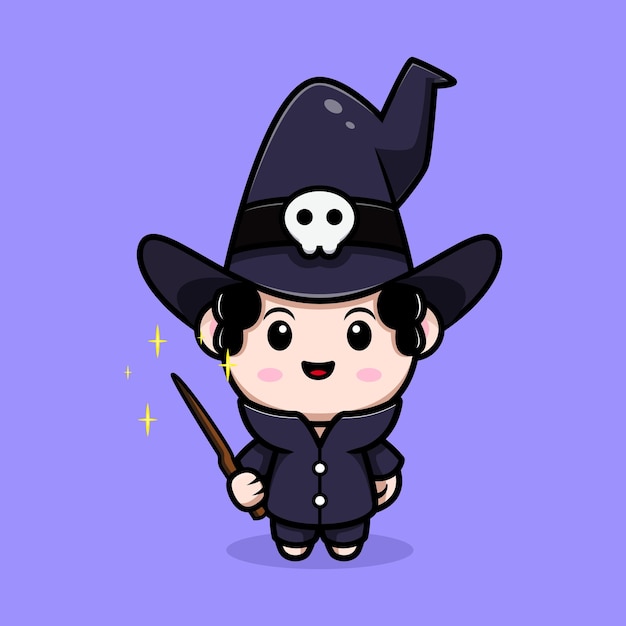The image is a cartoon-style drawing of a little boy standing in front of a light lavender purple background. The central character is depicted with a white face, pronounced black eyes, and a smiling mouth, complemented by two rosy cheek prints. He dons a deep, darker purple pointed brimmed hat, which features a black band decorated with a simple skull emblem—comprised of two eyes but no mouth, maintaining a non-horror, cartoonish appearance.

The boy is dressed in a small, black magician’s or wizard’s outfit, characterized by a high-neck tunic that is buttoned up with two prominent buttons. In his hand, he holds a magical wand emitting small yellow stars, adding to the charming, whimsical theme of the drawing. The overall style is front-facing, with the character engaging the viewer directly, and the artwork has an anime-inspired feel, emphasizing the fantastical and playful elements, potentially suitable for a holiday setting.